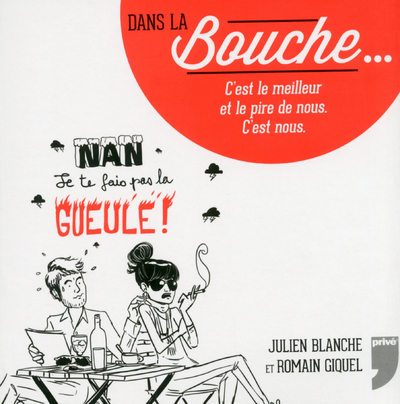The image depicted is a French advertisement featuring a detailed and expressive illustration. Dominating the upper left corner is a large red semi-circle partially cut off by the top right corner, containing prominent black and white text. The text reads "Dans La Bouche," with "Bouche" in large white letters and "Dans La" in black, followed by the phrases "C'est le meilleur et le pire de nous. C'est nous." Below this, the illustration portrays a man and a woman seated at a table in a black and white sketch style. The woman, with dark hair and wearing black sunglasses, is smoking a cigarette, while the man appears anxious, with sweat beads on his forehead, holding a document. The table in front of them features a wine bottle, glasses, and a cup with a spoon. Above the couple, black letters frosted with snow spell out "Nan," followed by "Je t'ai fait pas la gueule!" in cursive and fiery red letters. Small black storm clouds surround the text, adding to the tension of the scene. At the bottom left corner are the names "Julian Blanche, Romain, Seagal," and a pair of names are also noticeable at the bottom right, along with a large gray apostrophe. This intricate composition conveys a dramatic and emotional narrative through its vivid artwork and evocative text.